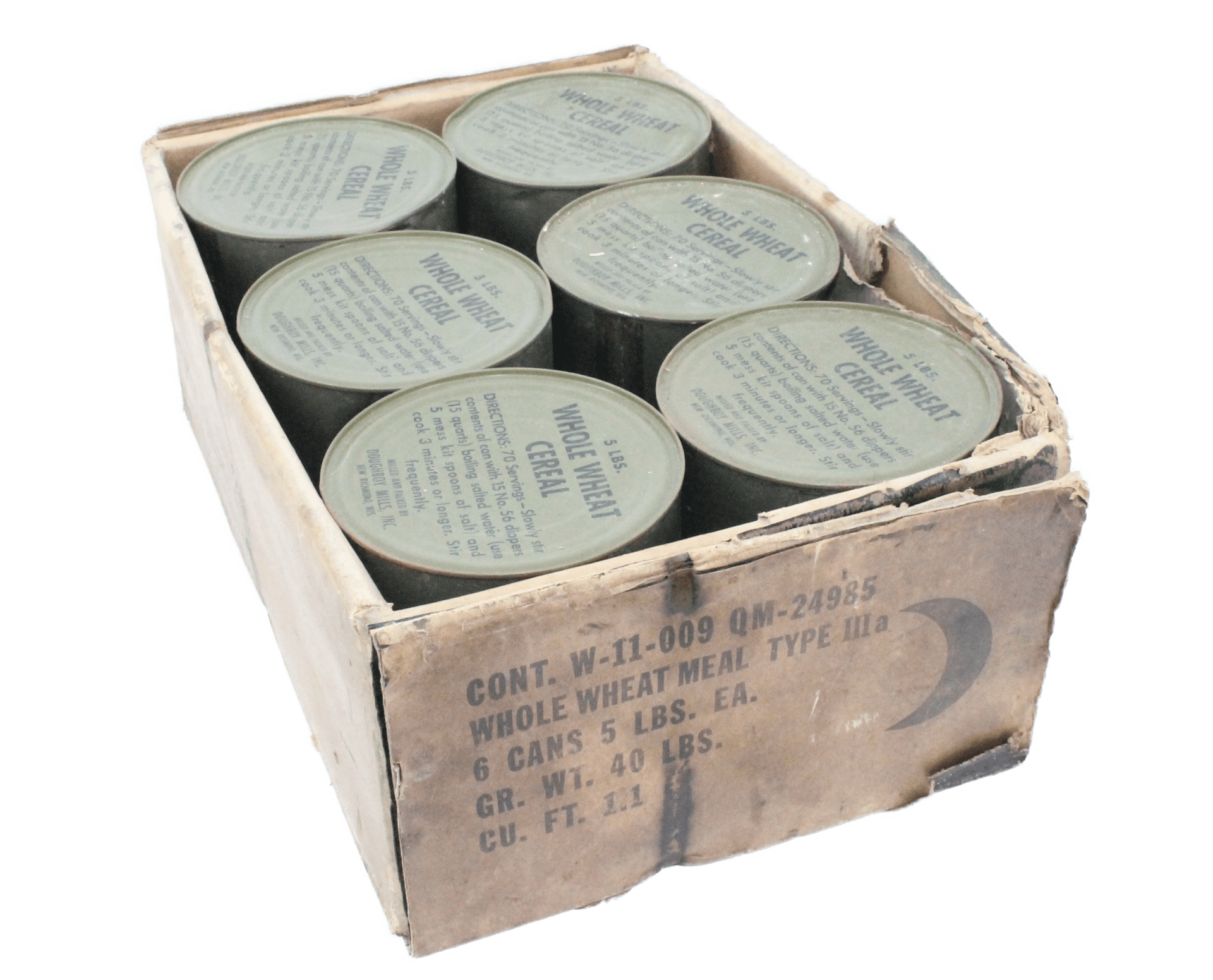This photograph captures a weathered and aged cardboard box, once used for packaging whole wheat cereal. The box is rectangular in shape and notably lacks a lid. Constructed of particularly thick cardboard, its exterior has faded over the years to a nearly gray hue, hinting at its long history. 

On the front, black lettering painstakingly lists the contents: 

- "CONTENTS W-1009 QM-24985"
- "Whole Wheat Meal Type III (Roman numerals), a6 Cans"
- "6 Cans, 5 Pounds Each"
- "Gross Weight: 40 Pounds"
- "Cubic Foot: 1.1"

A crescent moon symbol adorns the right side, adding a unique touch to the otherwise utilitarian design. Within the box, all six steel cans of whole wheat cereal are still present. Each can is marked "5 Pounds Whole Wheat Cereal" along the top. Although the cans feature usage directions, the text appears too faded to decipher clearly. The overall appearance of the box and its contents suggest significant age and use, giving it a historical and nostalgic essence.